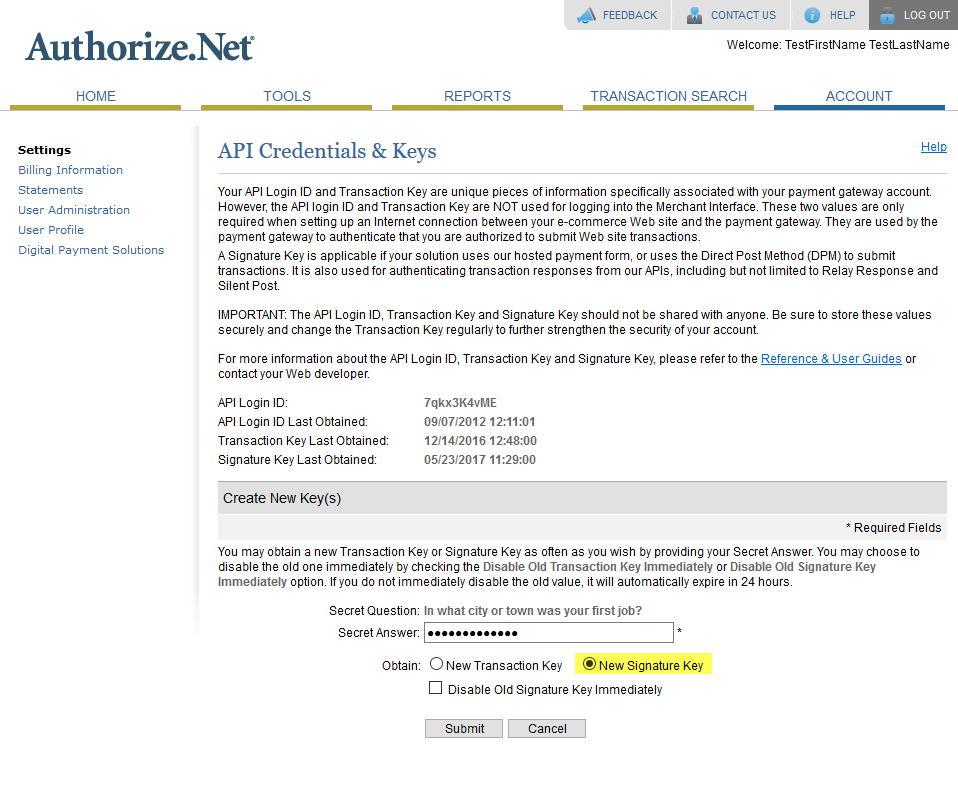This image is a well-organized screenshot of an Authorize.net webpage, primarily focused on text. At the top of the page, "Authorize.net" is prominently displayed in large, dark blue letters. In the upper right corner, there is a gray rectangular menu with options for "Feedback," "Contact Us," and "Help," ending with a black rectangle that reads "Log Out." Beneath this, a message welcomes the user identified as "Test First Name Test Last Name."

Just below the Authorize.net header, there are five rectangular navigation buttons labeled "Home," "Tools," "Reports," "Transaction Search," and "Account." On the left side of the page, a menu column lists various options: "Settings," "Billing Information," "Statements," "User Administration," "User Profile," and "Digital Payment Solutions."

The main content of the page discusses API credentials and keys in detail. It explains that the API login ID and transaction key are unique identifiers specific to a user’s Payment Gateway account. It clarifies that these credentials are used to authenticate payments and set up an Internet connection between the e-commerce website and Payment Gateway, rather than for logging into the merchant interface.

A highlighted paragraph emphasizes the importance of keeping the API login ID, transaction key, and signature key confidential. This section cautions users not to share these critical pieces of information. Following this is a detailed technical explanation of the API login ID, transaction key, and signature key, accompanied by a series of numbers for reference.

The page also provides options for managing these keys. Users can create a new key and are guided through the process of obtaining a new transaction key. This includes filling in a secret answer for added security, shown as a series of dots. At the bottom of the page, users can choose to obtain a new transaction key or disable the old signature key immediately, with options to "Submit" or "Cancel."